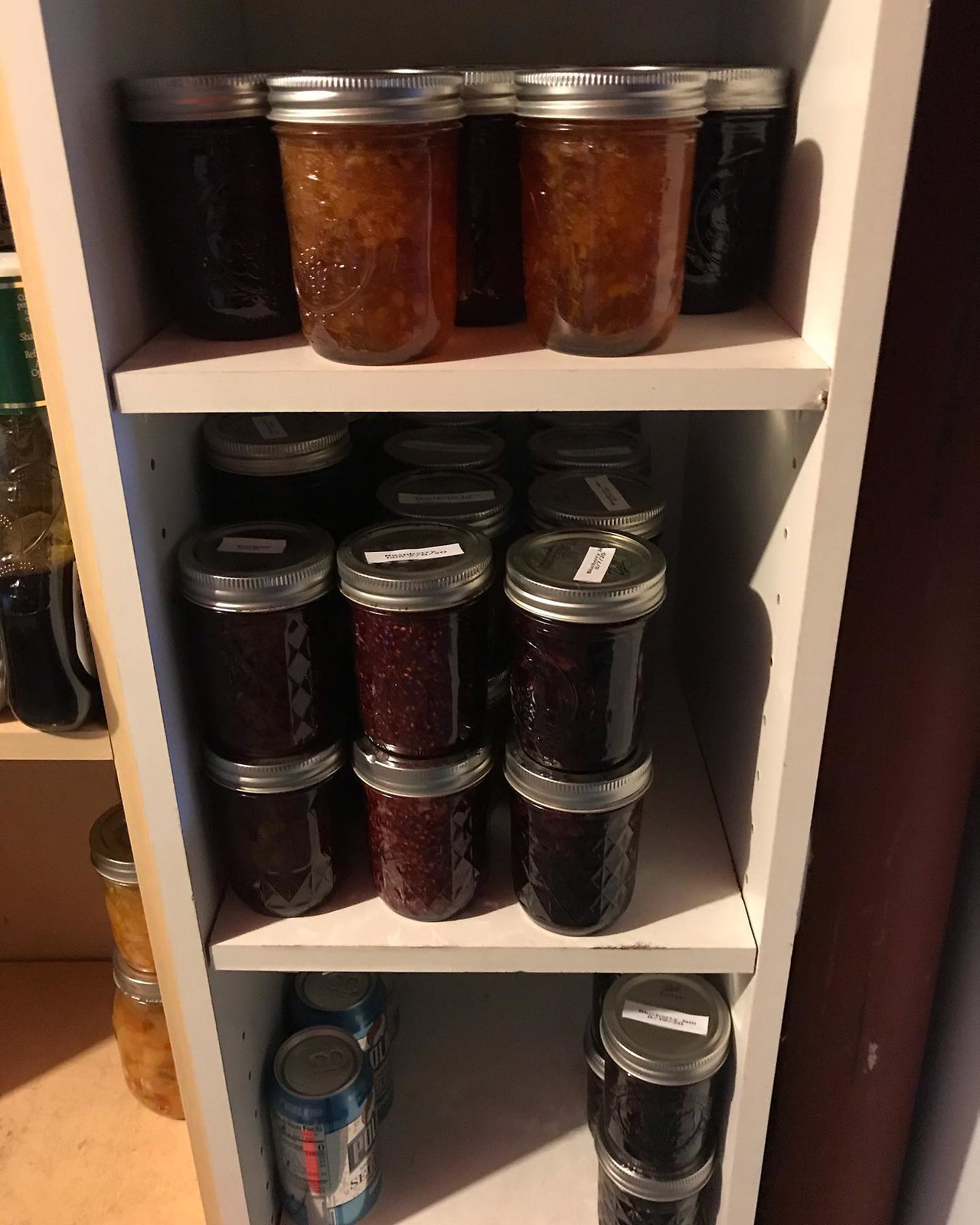This image depicts a tall, rectangular white cabinet, partially cut off at the top, revealing three visible shelves filled with an array of jars and cans. Each shelf holds a variety of items in neatly organized rows. The middle shelf, notable for its greater height, accommodates two tiers of jars, totaling approximately 18 jars arranged in three rows. These jars appear to be filled with preserved food items, such as jams or jellies, and feature silver lids with white labels. The bottom shelf contains a mix of items, including blue and silver cans, with one showing the partial label "P-O-L." Additionally, mason jars with various labels and contents are present, including ones that look like peach, raspberry, blueberry, and grape jams. The upper shelf also holds jars, some containing orange preserves with visible chunks. The overall scene suggests a well-stocked pantry within a home, meticulously organized for easy access to homemade preserves.